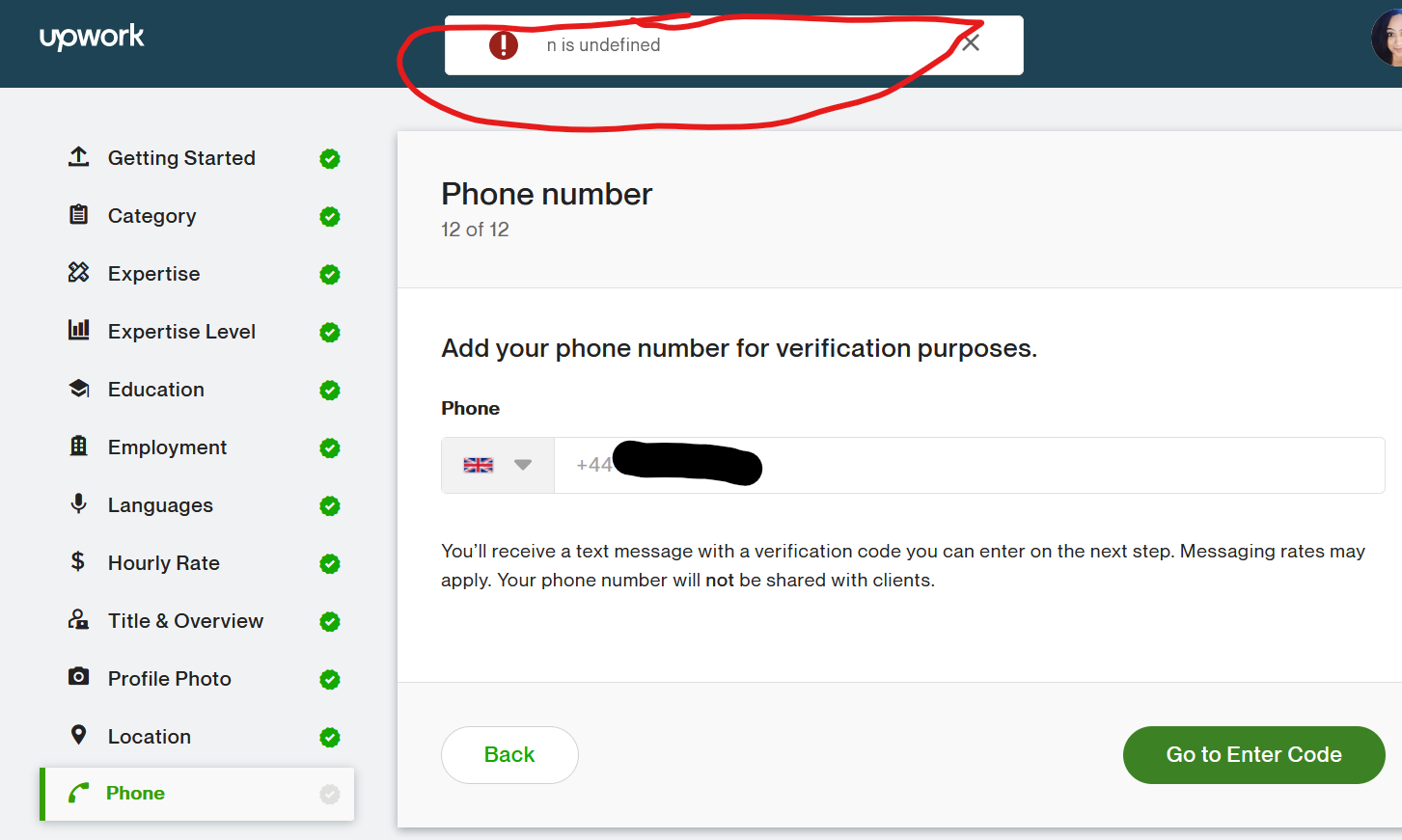The image features a light blue background with a prominent black header at the top displaying the Upwork logo. Centered within this header is a search box surrounded by a bold red outline, indicating an issue. Inside the search box, there is a red circle with an exclamation point, labeling it as "undefined" with an 'X' icon at the end. Adjacent to this, there is a semicircle showing a partial profile picture of a person. 

Below the header, the light blue background continues, listing various profile sections including "Getting Started," "Category," "Expertise," "Expertise Level," "Education," "Employment," "Languages," "Hourly Rate," "Title and Overview," "Profile Photo," and "Location." Each category has a green circle with a checkmark, signifying their completion.

At the bottom of the image, there is a box outlined with a green line on the left. Inside this box, there is an icon of a phone and the text "Phone." To the right, it states "Phone number 12 of 12," encouraging the user to "add your phone number for verification purposes." It includes a partially visible British flag icon with a down arrow and the country code "+44," with the rest of the phone number blacked out. Below, there's a message indicating that a verification code will be sent via text, stating, "Messaging rates may apply. Your phone number will not be shared with clients."

Finally, at the bottom left, there is a white "Back" button, and at the bottom right, a green "Go to Enter Code" button is present.